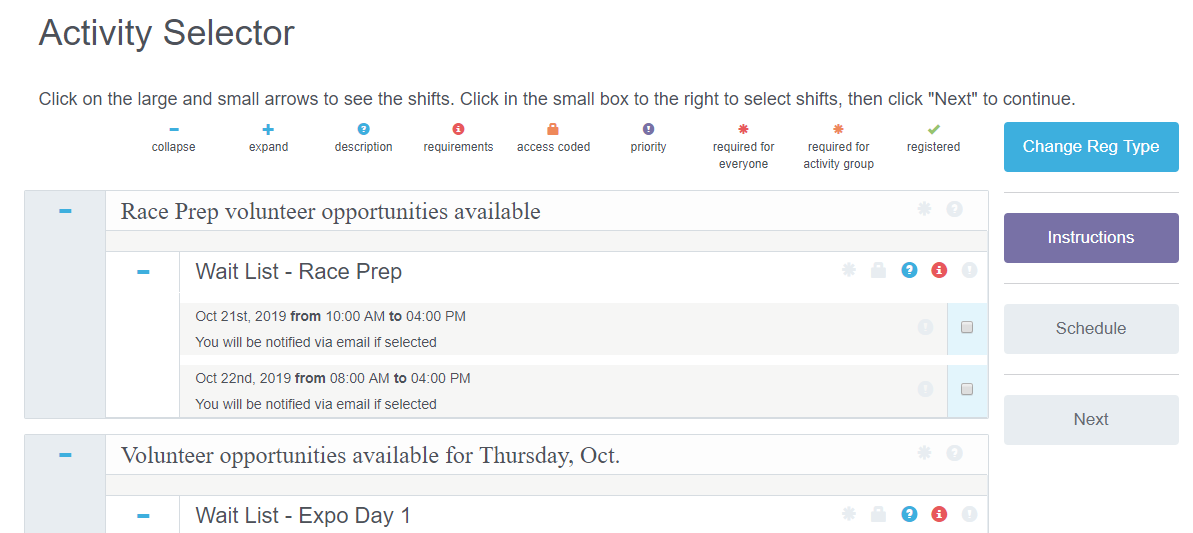This is a detailed caption of an image showcasing a landscape-oriented screenshot from a website, likely viewed on a laptop. 

---

The screenshot captures a webpage with a title "Activity Selector" positioned at the top-left corner. Directly below the title, there is an instructional text that reads: "Click on the large and small arrows to see the shifts. Click in the small box to the right to select shifts, then click next to continue."

Beneath this instructional text, a series of icons with their corresponding labels are aligned horizontally. From left to right, the icons include:

1. A minus sign labeled "Collapse."
2. A plus sign labeled "Expand."
3. A question mark labeled "Description."
4. A letter "I" icon labeled "Requirements."
5. A lock icon labeled "Access Coded."
6. An exclamation mark labeled "Priority."
7. A red asterisk labeled "Required for Everyone."
8. An orange asterisk labeled "Required for Activity Group."
9. A green check mark labeled "Registered."

Following the icons, two separate tables are displayed. The first table, titled "Race Prep Volunteer Opportunities Available," lists several race prep options, including a section for a "Waitlist Race Prep." The second table, positioned directly below the first, is labeled "Volunteer Opportunities Available for Thursday, October" and includes multiple options, such as "Waitlist Expo Day One."

On the right side of the screenshot, four vertically stacked buttons are visible. The top button is blue with white text reading "Change Reg Type." The second button is purple with white text reading "Instructions." The third and fourth buttons, labeled "Schedule" and "Next" respectively, both have gray backgrounds with black text.

This detailed description ensures a comprehensive understanding of all visible elements in the webpage screenshot.